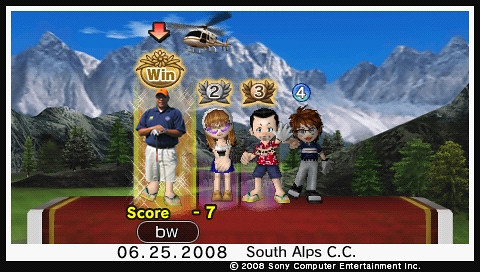Screenshot from a video game featuring a UI overlay with various text and images. In the lower right-hand corner, a black border contains the text "Copyright 2008 Sony Computer Entertainment Incorporated." Above this text, a white line displays "06.25.2008 South Alps, C.C." A small capsule-shaped image with lowercase "bw" is also present. The word "SCORE" appears in yellow with a score of '-7'.

The main image showcases a man dressed in a blue button-down shirt, orange golfer's hat, white shorts, and flip-flops. The word "WIN" is displayed above him. Surrounding this man are three cartoon figures. The first figure (number 2) is a girl with brown hair, purple glasses, a blue skirt, and tan shoes. The second figure (number 3) is a boy with black hair, a red shirt, blue shorts, and flip-flops. The third figure (number 4) appears to be an older lady, despite being the same height as the children, featuring brown spiky hair and glasses.

In the background, there is a picturesque landscape of snowy mountains and a bright blue sky, with additional mountain ranges and pine trees below. Almost at the center of the image, a helicopter is seen flying. The overall scene effectively combines real photographic elements with animated characters in a mountainous alpine setting.